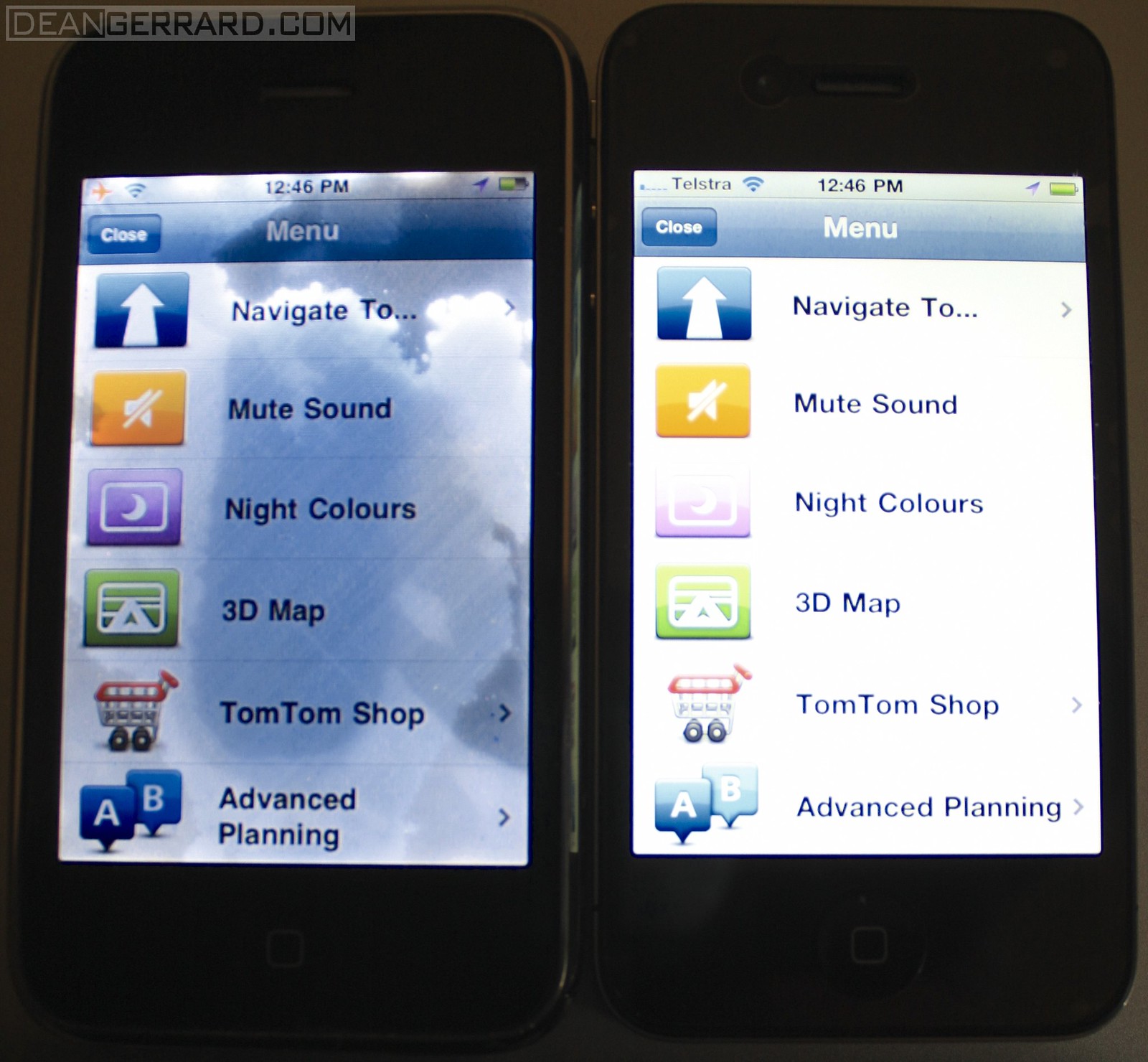This detailed photograph features two identical smartphones resting side-by-side on a possibly hidden surface, with their screens illuminated to display the same navigation menu at 12:46 PM. The device on the left has a dimmer screen compared to the brighter one on the right. Both screens exhibit the following menu options: "Navigate to" accompanied by an up arrow icon, "Mute sound" indicated by a speaker icon, "Night colors" shown with a moon icon, "3D map" with a 3D map icon, "TomTom shop" represented by a shopping cart icon, and "Advanced planning" denoted by a logo featuring the letters 'A' and 'B'. Notably, the upper left-hand corner of the photo includes the watermark "DeanDeanGirard.com," and the framing of the photograph tightly focuses on the phones, making the underlying surface indiscernible.